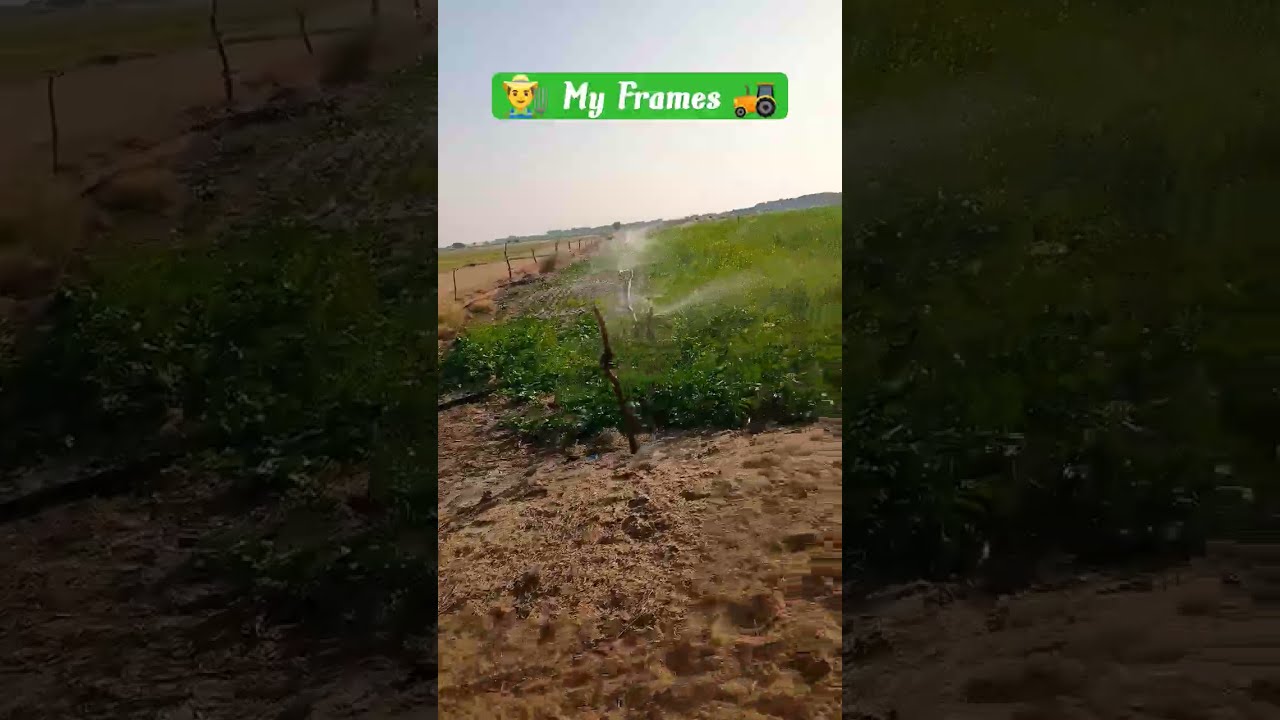The image is divided into three vertical sections, with the middle section featuring a bright photograph of a sunlit farm field. Most of the field is lush with green plants, and automatic sprinklers are actively spraying water over the crop. In the foreground, the ground is covered with brown soil transitioning into an unkempt patch of dry grass. On the left side of the field, there is a brown pathway that appears to be fenced, possibly intended for farming activities. The top quarter of the photo showcases a clear, light blue sky. The left and right sections of the image contain darkened, underexposed close-ups of their respective sides from the central section. Overlaying the top part of the image are the words "My Frames," flanked by a farmer emoji on the left and a tractor emoji on the right, giving a playful touch to the photograph's presentation.